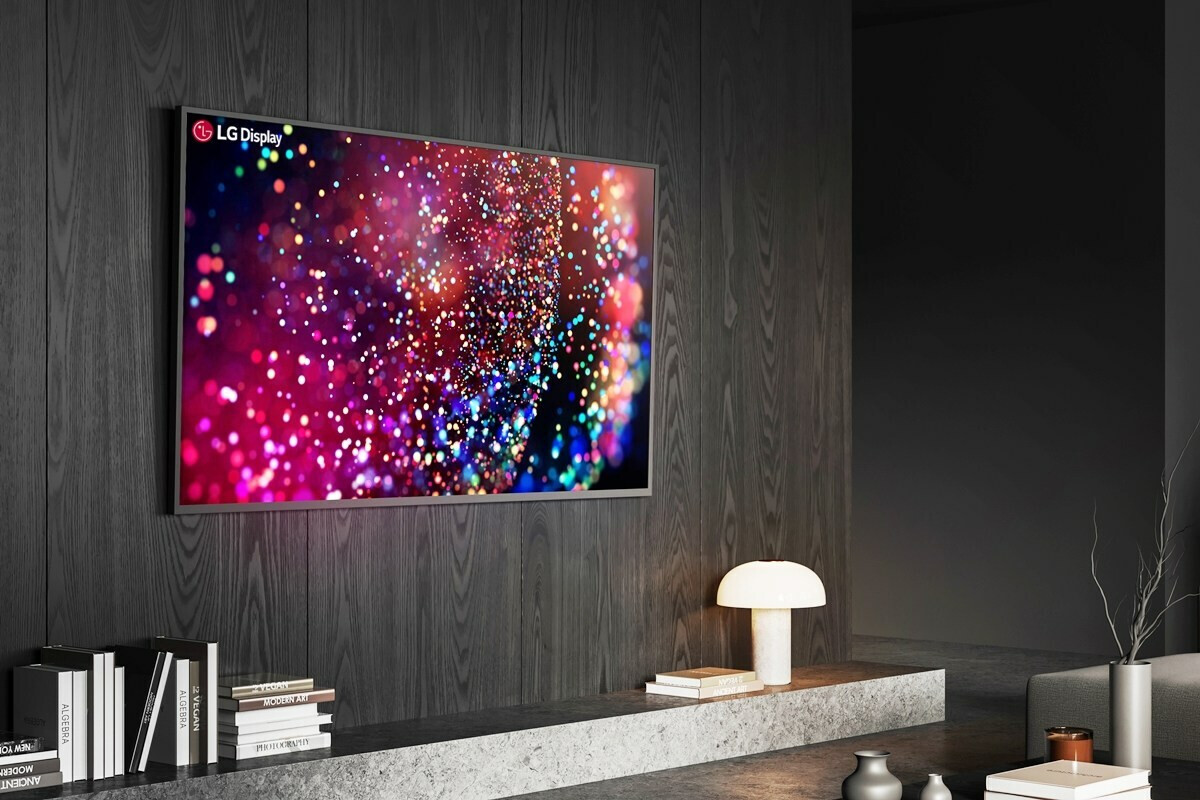The image is a color photograph in landscape orientation, showcasing the interior of a modern room. The focal point is a flat-screen TV mounted on a wall made of dark gray and tan wood panels. The TV, identified as an LG display from the logo and text on the top left corner, is showcasing a colorful screensaver composed of multi-colored dots and a hazy background primarily in shades of blue, green, and pink, creating the effect of a dynamic light show.

Below the TV, a low-lying bookshelf holds an assortment of books on its left side and features a distinctive white, mushroom-shaped lamp on the right. The floor appears to be a brownish cement type, contributing to the room's minimalist aesthetic.

To the right of the bookshelf, several vessels rest directly on the floor, accompanied by a small white table or pedestal. To the left, a gray cylinder filled with branches adds an organic touch to the setting. Further to the left, parts of a small couch and the baseboard, transitioning from dark black to gray, are visible, completing the modern and cohesive decor of the room.